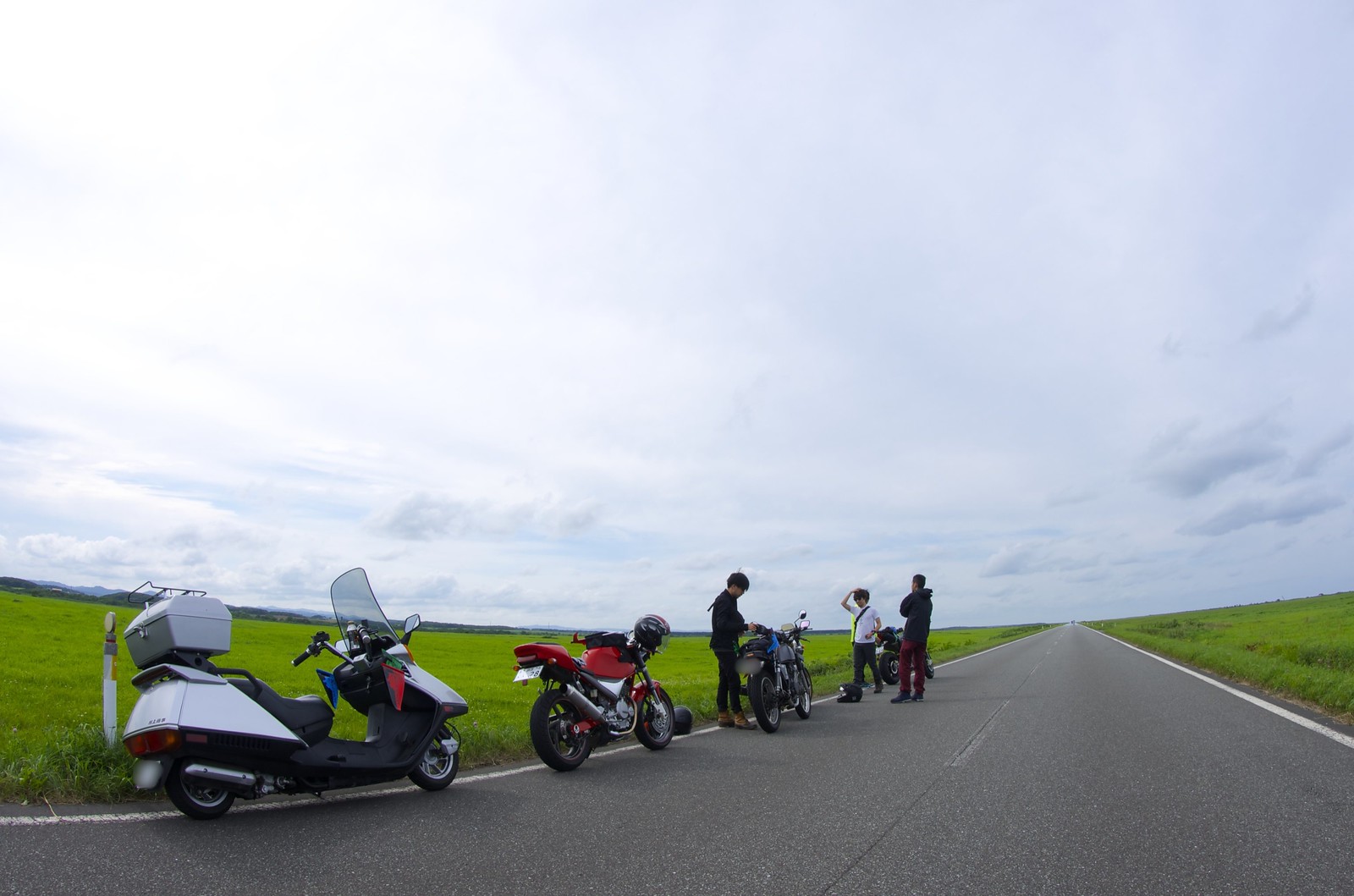In this image, we see a group of people who have pulled over their motorbikes on a long, straight, asphalt road that stretches to the horizon, flanked by vast fields of green on both sides. The foreground features four motorbikes parked on the road's left side. Closest to the camera on the lower left is a white scooter with a black seat and a gray storage container on the back, plus a large windshield. In front of the scooter is a red motorcycle with a helmet hanging from its handlebars. The third motorbike, primarily black with blue accents, has a man dressed in black with brown shoes standing to its left, looking down. The fourth motorbike is less visible, partially obscured by two men in front of it—one wearing a white shirt and black pants, the other in red pants and a black shirt. A black helmet lies on the ground near them. A flash of fluorescent yellow clothing is barely visible behind the fourth bike. To the immediate right of these men is another individual, hinting at another unseen motorbike. The scene is framed by white side lines and a faded dashed center line, marking it as a two-way road beneath a bright but cloud-filled sky.